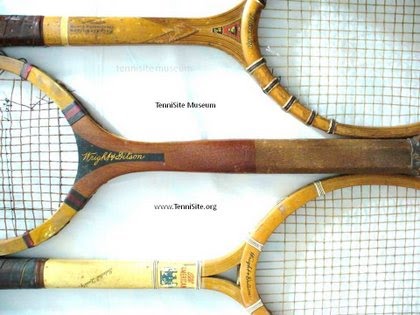This photograph showcases a trio of antique wooden tennis rackets placed against a white background. The rackets are arranged with two handles pointing to the left and the middle one's handle pointing to the right, creating a visually intriguing pattern. Each racket has its own distinct characteristics: the top racket features a dark handle transitioning into a light golden wooden frame, the middle racket is made of darker wood with reddish-brown tones and dark and red stripes around its head, and the bottom racket boasts a dark handle with a yellow shaft leading to a light wooden frame. The strings on each racket are evident and add to their antique appearance. The setup appears to be on a table or possibly a wall, captured from a top view. Between the rackets, textual elements are present, stating "Tennis Site Museum" along with a watermark, "www.TennisSite.org."